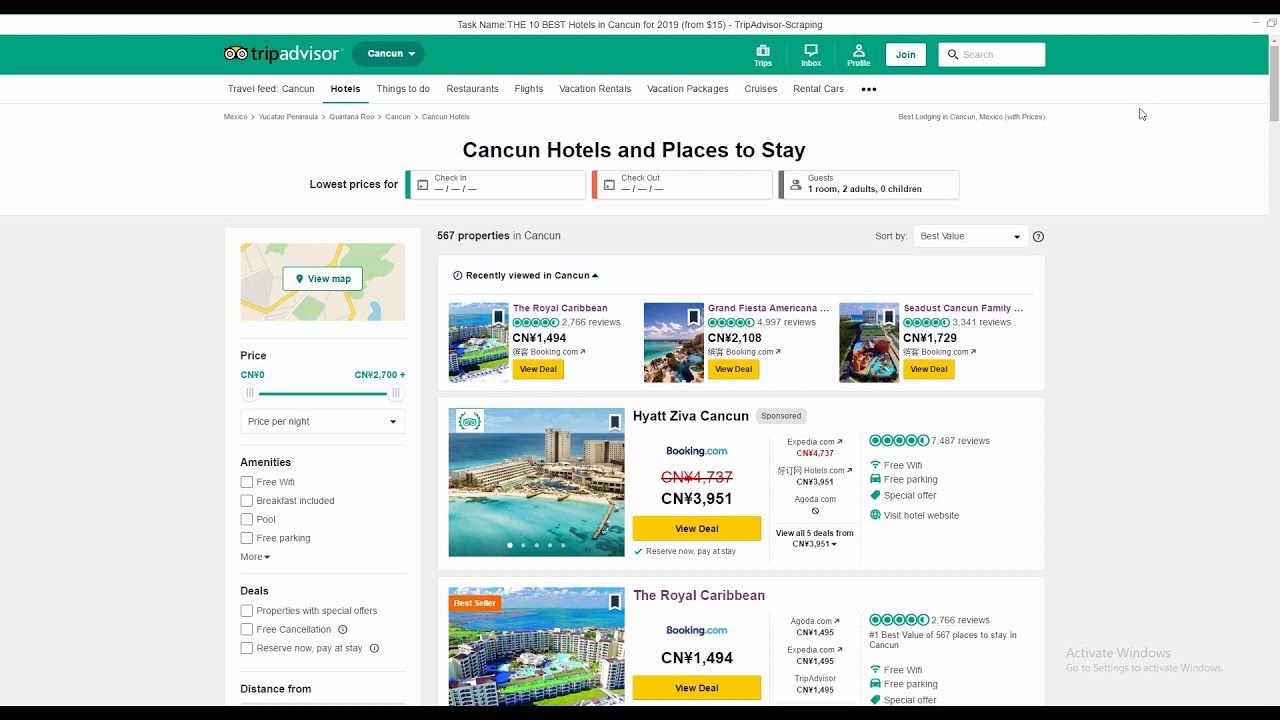This screenshot, taken from the TripAdvisor website, prominently features the TripAdvisor logo and name on a green bar at the top. Beneath the logo is a series of closely packed tabs, though the text is too small to discern their exact labels. On the left-hand side of the screenshot, a comprehensive set of filtering options is displayed, allowing users to refine their search according to various trip criteria. The main section of the webpage is dedicated to showcasing Cancun hotels and places to stay. It includes interactive fields to input the check-in and check-out dates and specify the location more precisely. The central section of the screen shows search results, which currently list two accommodation options along with their respective prices, offering a glimpse into potential vacation choices.